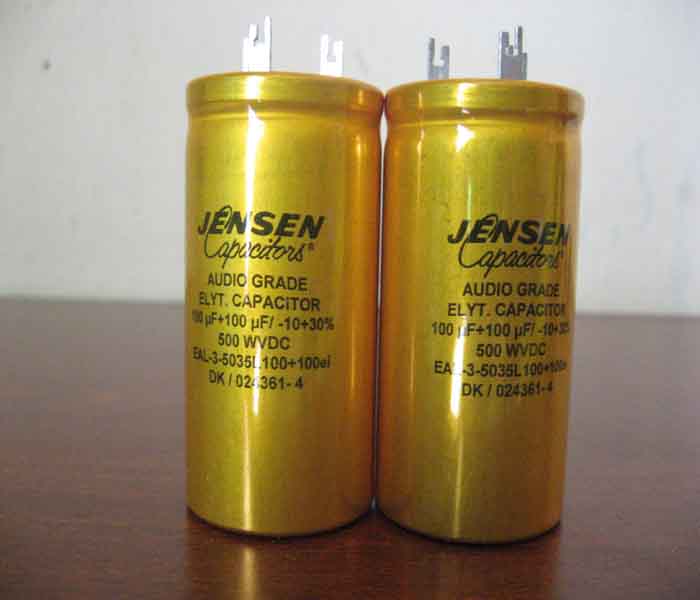The photograph features two metallic cylindrical objects with a shiny gold finish, resting on a dark wooden table. These objects, which are about the size of a Coke can, have pairs of metal prongs protruding from their tops, indicating they are designed to be plugged into an electronic device. Each cylinder is labeled prominently with "Jensen capacitors" in bold black print and script text. Beneath this, the labels include technical specifications: "Audio Grade ELYT capacitor" followed by "100 PF, ±10%, ±30%, 500 WVDC." Additional details include various alphanumeric codes and percentage values, some of which are partially obscured by reflections. Behind the table, the background displays a plain white-gray wall, occupying about half of the photo's vertical space. The lighting in the image highlights the reflective surfaces of the capacitors, emphasizing their bright gold color. The overall scene is tightly framed, directing focus towards the capacitors and their detailed labeling.